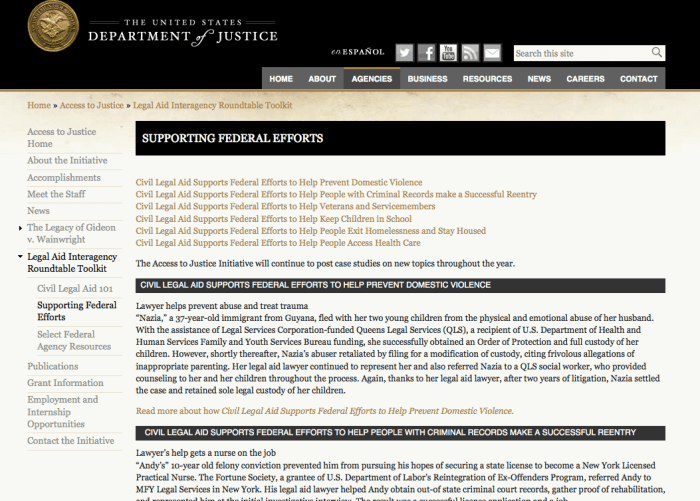This detailed description offers a comprehensive view of a webpage from the United States Department of Justice. Here's a cleaned-up and formatted version to use as a descriptive caption:

---

**Detailed Overview of a United States Department of Justice Webpage**

The image showcases the header of a webpage from the United States Department of Justice. Centered at the top, the header features white text reading, "The United States Department of Justice." To the left of this text is a golden coin emblem. Right-aligned in the header are navigation tabs including: Home, About, Agencies, Business, Resources, News, Careers, and Contact.

Above the header, a search bar prompts users to "Search this site," flanked by social media icons for Twitter, Facebook, YouTube, RSS feeds, and email.

Below the header, the background shifts to a slightly white hue. Prominently displayed is the phrase, "Supporting Federal Efforts." The section beneath it, written in brown text, details various initiatives under "Civil Legal Aid," aimed at supporting federal efforts. The initiatives listed are:
- Prevent Domestic Violence
- Help People with Criminal Records Make a Successful Reentry
- Help Veterans and Service Members
- Help Keep Children in School
- Help People Exit Homelessness and Stay Housed
- Help People Access Healthcare

Further down, black text notes, "The Access to Justice Initiative will continue to post case studies on new topics throughout the year."

At the bottom of the section, another text emphasizes "Civil Legal Aid" and its role in supporting federal efforts to prevent domestic violence. It then narrates the story of Nazla, a 37-year-old from Guyana who escaped the abuse of her husband. With assistance from Queens Legal Services (QLS), funded by the U.S. Department of Health and Human Services Family and Youth Service Bureau, she obtained an order of protection and full custody of her children. Despite her abuser’s retaliatory legal maneuvers, Nazla’s legal aid lawyer and a QLS social worker provided continuous support. After two years of litigation, she achieved sole legal custody of her children.

Lastly, users are encouraged to "Read more about how Civil Legal Aid supports federal efforts to help prevent domestic violence," with additional navigation options on the left side of the page. These options include: Home to Access to Justice Home, About the Initiative, Accomplishments, Staff News, The Legacy of Gideon, Legal Aid, Interagency Roundtable Toolkits, Civil Legal Aid 101, Supporting Federal Efforts, Supporting Federal Agency Resources, Publications, Grant Information, Employment and Internship Opportunities, and Contact the Initiative.

---

This description provides a clear and structured overview of the webpage, highlighting key elements and their significance.